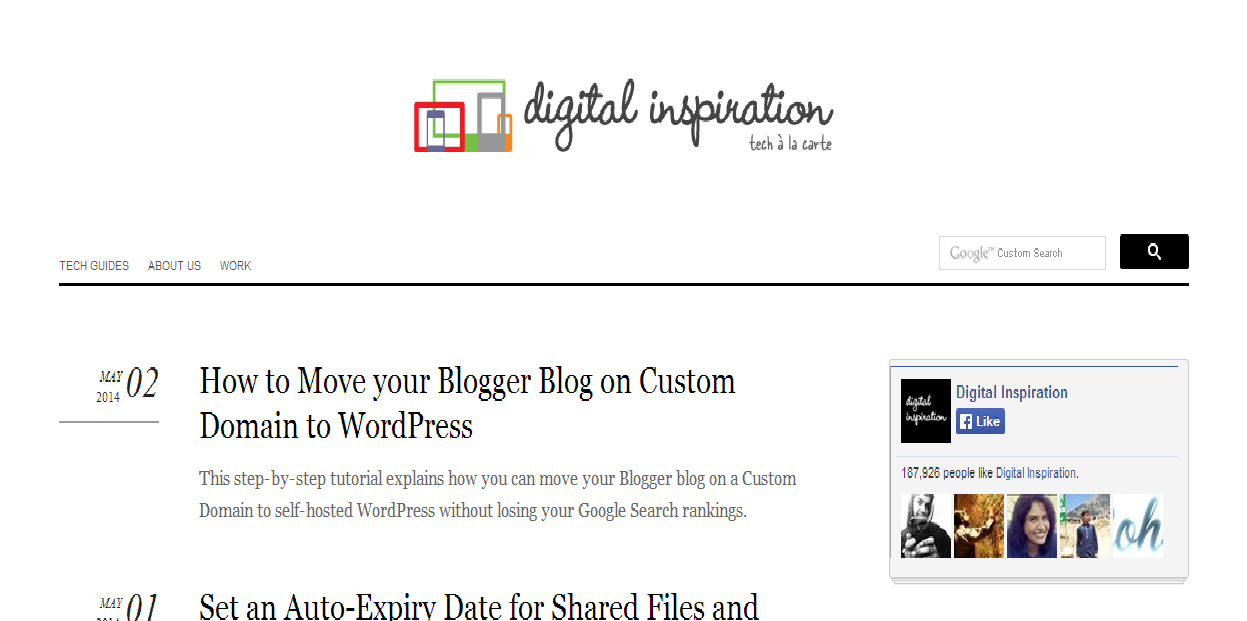**Digital Inspiration Tech Alakati Overview**

The top section of the image prominently displays the heading "Digital Inspiration Tech Alakati" in bold, black text. Beneath this heading, on the left side, there is an icon featuring a variety of smartphone and tablet silhouettes in green, red, dark blue, gray, and orange hues.

The main webpage is shown directly below, featuring a vertical navigation panel on the left side with tabs labeled "Tech Guides," "About Us," and "Work." On the top right corner of the page, there is a search box accompanied by a black search button. 

On the main content area of the webpage, the date “May 2, 2014” is displayed on the left. The primary article heading reads, "How to Move Your Blogger Blog on Custom Domain to WordPress." This detailed, step-by-step tutorial explains how one can transfer their Blogger blog on a custom domain to a self-hosted WordPress site without negatively affecting their Google search rankings. 

Below this article heading, another date stamp “May 1, 2014” leads into a brief snippet titled, "Set an Auto Expiry Date for Shared Files," followed by a short introductory text.

To the right of the main content, there is a sidebar box labeled "Digital Inspiration" which features a blue Facebook Like button showing 87,000 likes and names 26 people as current followers. Beneath this information, there are profile pictures of five individuals.

The overall background of the image is white, providing a clean and structured layout for the web page content.